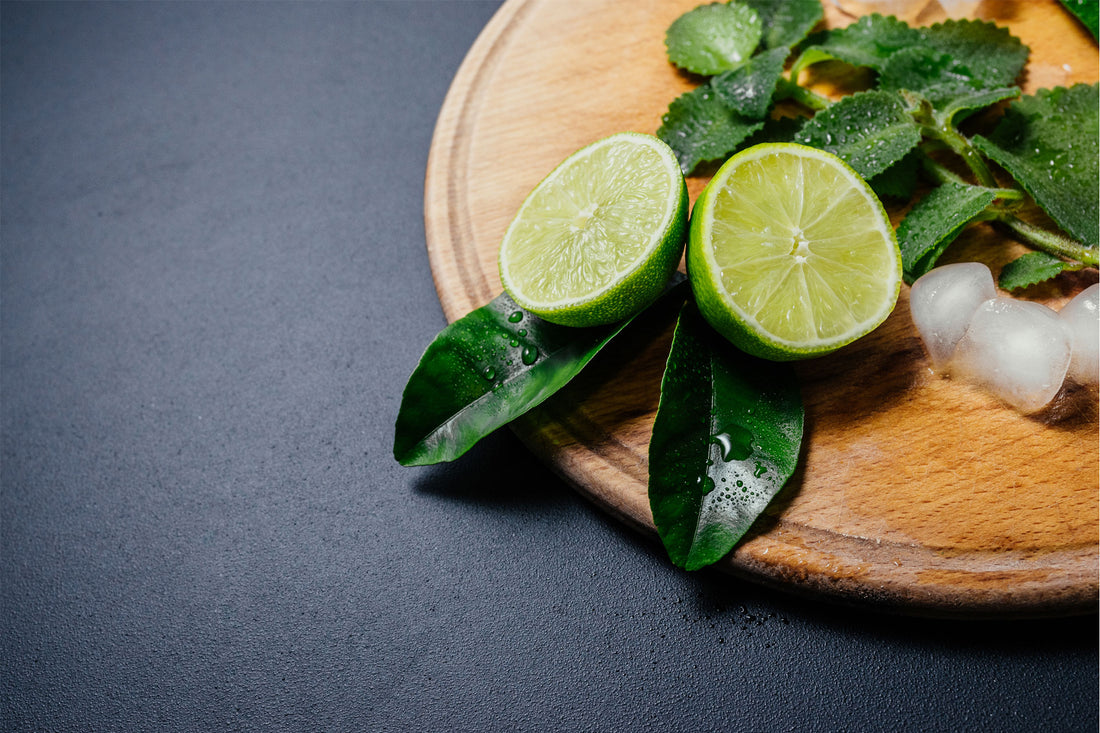This professionally lit stock photograph, taken indoors in a studio, features a meticulously arranged scene on a circular honey-gold wooden cutting board with a beveled edge. The main subjects on the board are several cold, watery green mint leaves, two halves of a fresh green lime, and a few strategically placed ice cubes. The background is a textured gray tabletop, partially obscured by droplets of water, enhancing the fresh and invigorating feel of the image. Only three-quarters of the cutting board is visible in the photo, suggesting a dynamic crop that draws the eye to the central elements. This image, perfect for use in restaurant menus or food advertisements, showcases professional lighting that avoids any harsh reflections or unwanted highlights.